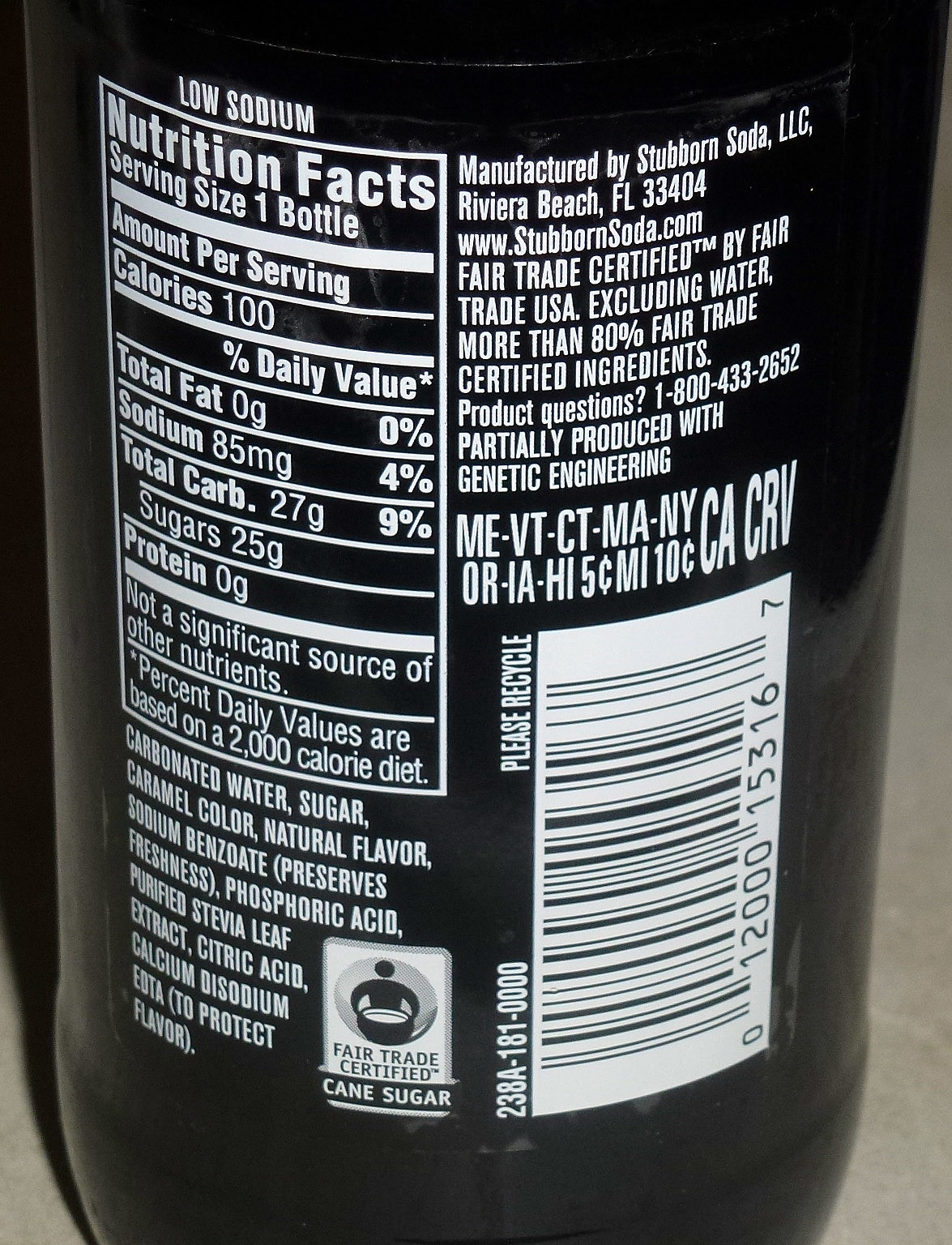The image is a colour photograph in portrait orientation, featuring a close-up of the back of a bottle, showcasing its label information. The bottle is dark, appearing black or possibly very dark brown, and could be made of glass or plastic. The label features white text on the dark bottle, making the information stand out clearly. The barcode is located in the bottom right corner, oriented vertically. Reflections running along the right side of the bottle, curving near the barcode, add a bit of glare that slightly obscures details.

In the top left corner, there is a portrait-oriented box labeled "Low Sodium" above the text "Nutrition Facts." Inside this box, it reads "Serving size: one bottle." Beneath this, in white capital letters, the ingredients are listed: "Carbonated Water, Sugar, Caramel Color, Natural Flavor, Sodium Benzoate (preservative), Phosphoric Acid, Purified Stevia Leaf Extract, Citric Acid, Calcium Disodium EDTA (to protect flavor)." Additional details indicate that the product is Fair Trade Certified with cane sugar.

The nutritional information: 100 calories, 0 grams of fat, 85 milligrams of sodium, 27 grams of carbohydrates (including 25 grams of sugars), and 0 grams of protein. At the top right of the label, it states "Manufactured by Stubborn Soda, LLC, Riviera Beach, Florida 33404." The bottle also encourages recycling and offers a number to call for questions. The background of the image is an off-white to gray tone, providing a neutral setting which helps the details on the bottle stand out.